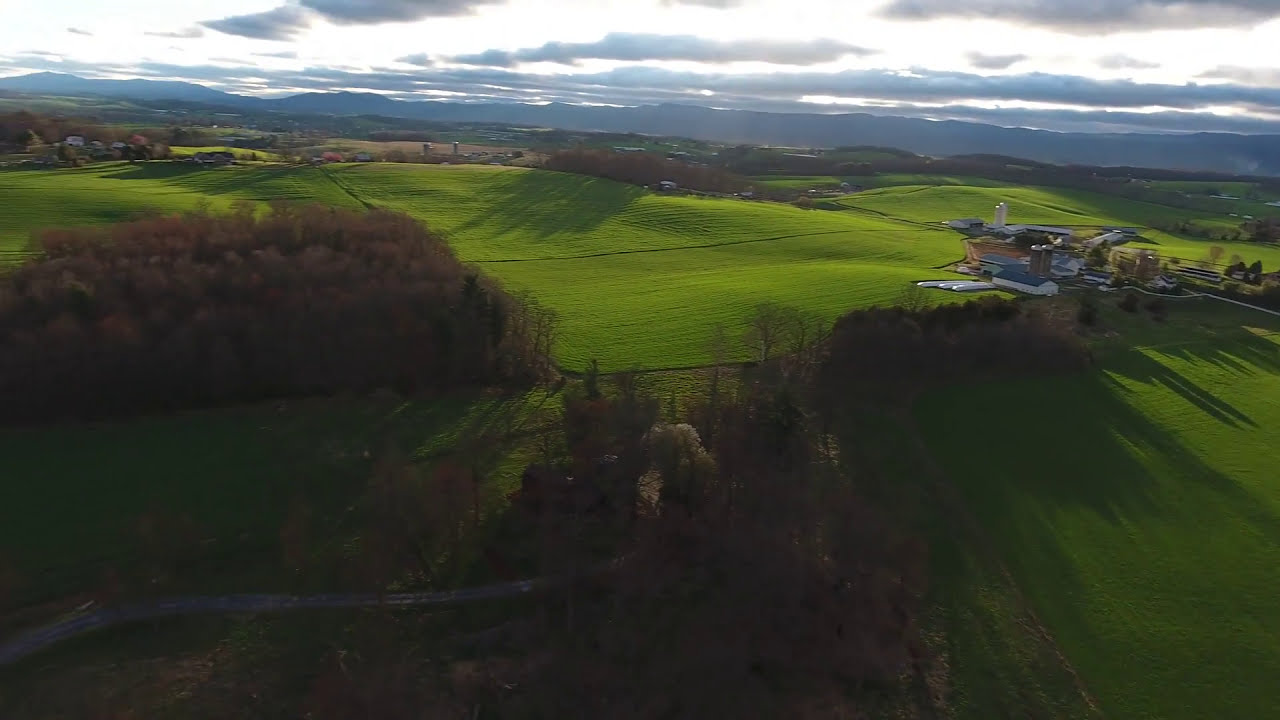This is an outdoor, aerial photograph set in the countryside, capturing a bright, sunlit landscape of rolling grassy hills and farmland. The image, a horizontal rectangle taken from a high elevation, showcases lush green fields interspersed with groves of brownish deciduous trees and large bushes. A winding road begins at the bottom left corner, curving upward and merging with the vegetation as it leads towards the central right part of the image, where a prominent farm with double silos and possibly greenhouses stands. Several other farms can be seen in the distance. The backdrop is defined by distant foothills or mountains, under a sky filled with gray clouds, with the sun casting a soft light indicative of either early morning or late afternoon. The colors in the photograph range from vibrant greens and browns to shades of gray, white, black, and beige, adding to the detailed and serene rural scene.